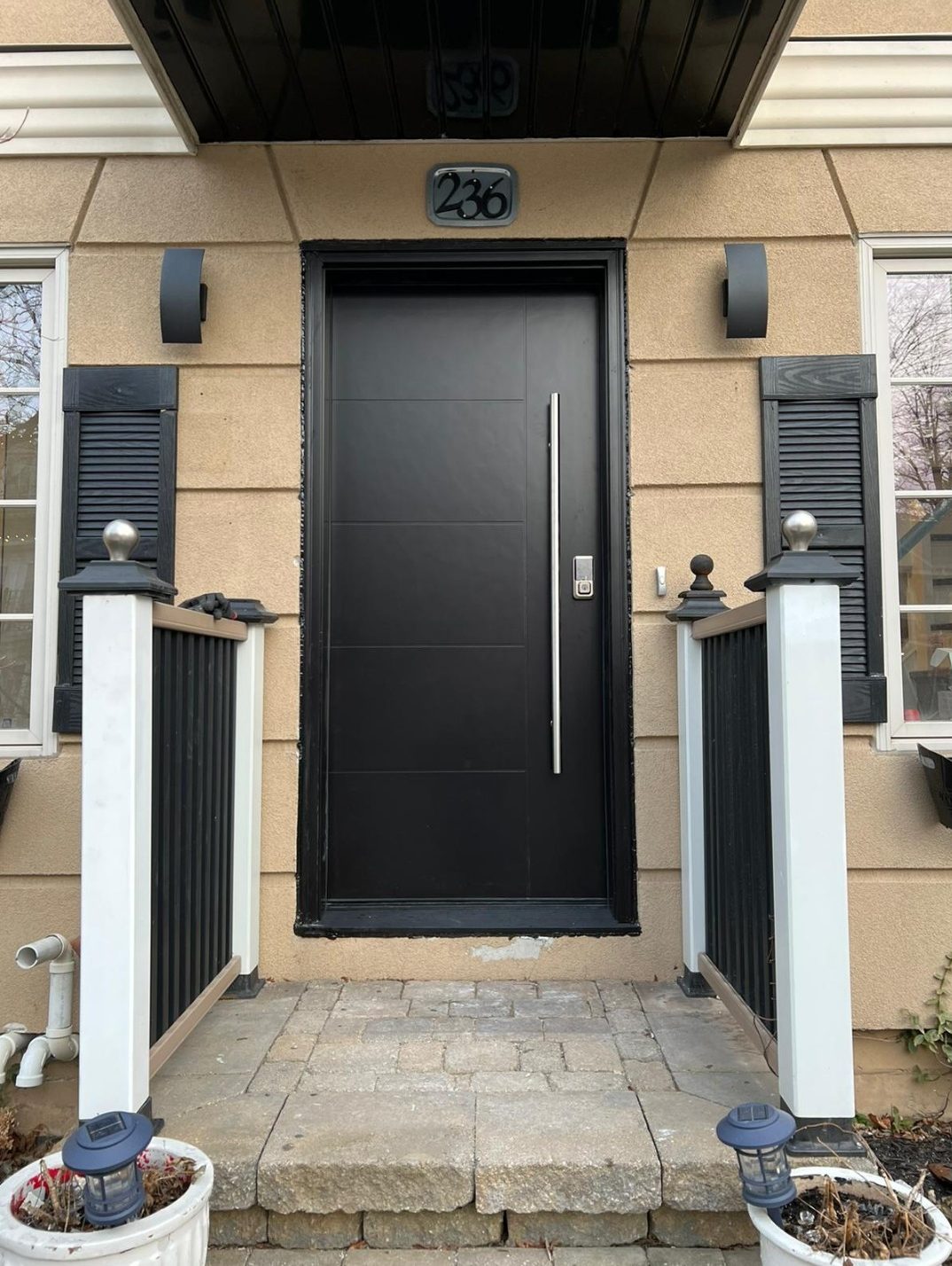In this outdoor daylight photograph, we are presented with a detailed, straight-on view of a house's front entrance. The house itself has a sandstone-colored exterior, contrasting with the jet-black front door, which features a stainless steel vertical door pull and matching silver handle and lock. Above the door is a silver plate displaying the house number "236" in black. The small, square front porch, approximately four by four feet in size, is made of cut stone. Flanking the walkway leading up to the door are railings with white posts topped with silver finials and black gates. On either side of the porch, there are white potted plants, unfortunately filled only with dirt and dead plants. Additionally, small lanterns are stuck into these pots. Adjacent to the door, partial views of white windows framed by black shutters are visible, adding to the symmetrical and tidy appearance of the house's entrance. An overhang above provides shelter from the elements.